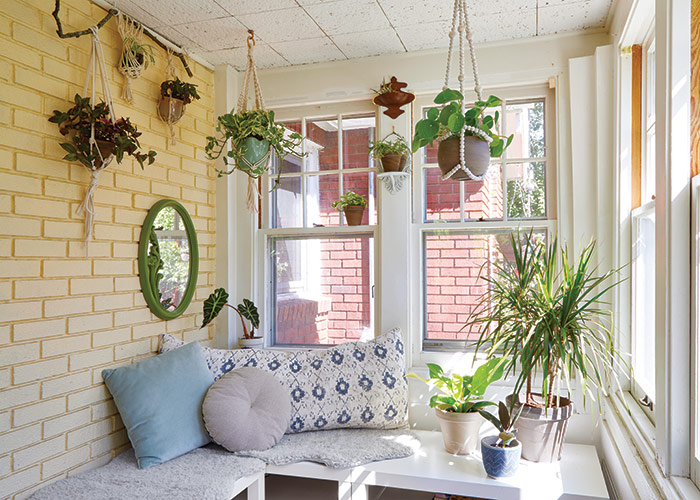The photo depicts a brightly lit sunroom with a cozy and inviting atmosphere. This enclosed veranda is adorned with cream and yellow-painted brick walls, featuring a prominent yellow back wall with a circular green mirror and several potted plants hanging from it. The ceiling has multiple hanging plant pots, adding lush greenery to the space.

White-framed large windows dominate two sides of the room, allowing sunlight to flood in and illuminate the interior. On the left side of the image, adjacent to the yellow brick wall, is a comfortable lounging area with cushioned seating, perfect for relaxation. The seating area includes white tables complemented by thick blankets and pillows, contributing to the room's warm and cozy ambiance.

In the background, through the windows, the front of a house with red brick walls can be seen, indicating that this sunroom is part of a larger home. The sunlight streaming through the windows enhances the bright and airy feel of the space, making it an ideal spot to enjoy sunny days indoors.